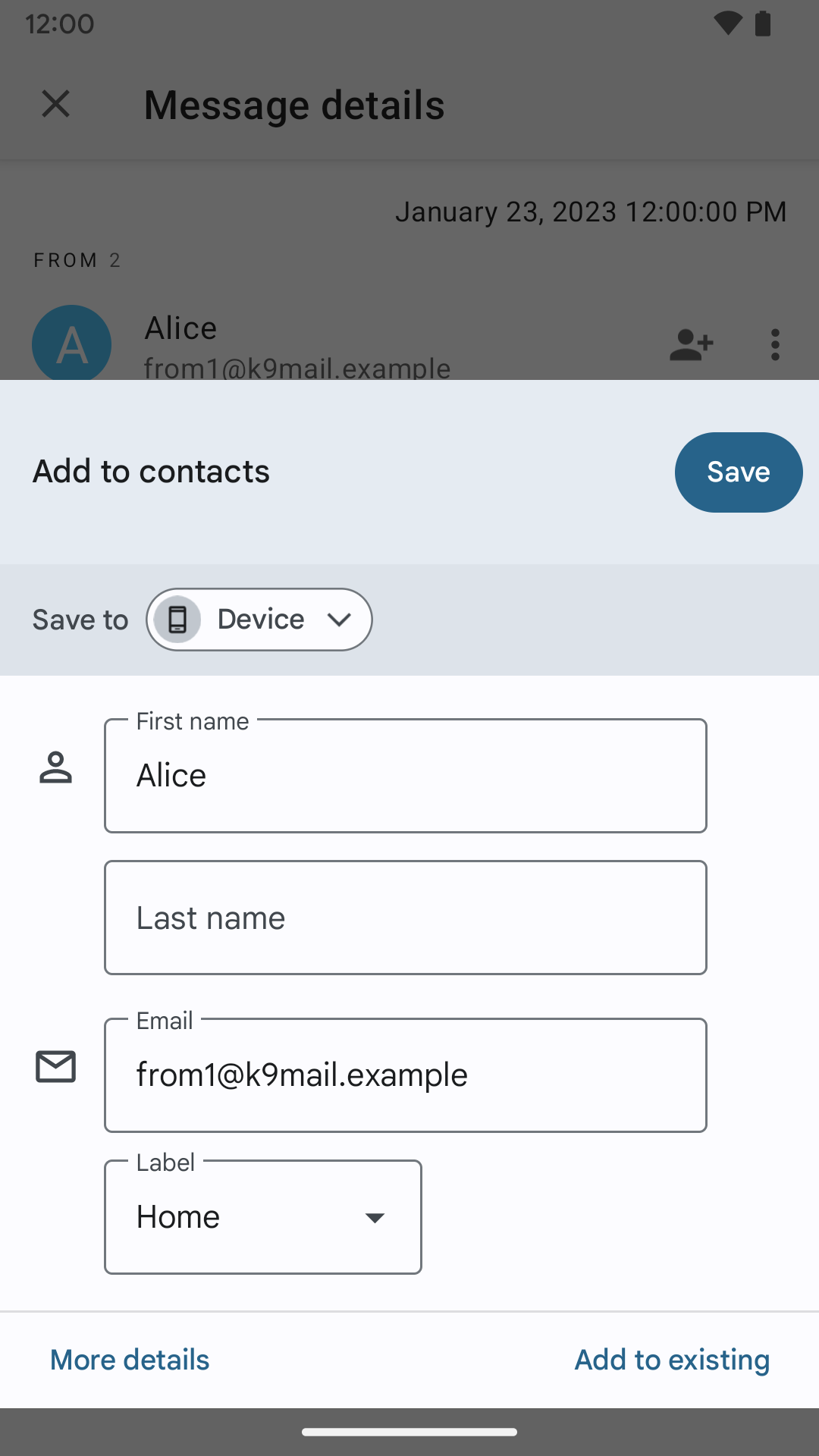This image is a screenshot taken from a mobile phone displaying an open pop-up menu. The background of the screen has a slight gray filter, visible only at the top. The status bar at the top shows the time "12:00 PM" on the left side, along with Wi-Fi and battery icons on the right.

Below the status bar, in black font, is a header that reads "Message details." The message timestamp is "January 23rd, 2023 at 12 PM" from a sender named Alice, with the email address "1atk9mail.example."

The main pop-up menu is white with an off-white top bar. This bar contains the text "Add contacts" in black font, and to the right, there is a purple oval button labeled "Save" in white text. Below the top bar, a darker gray rectangle with the label "Save to" in black font presents a dropdown menu, which currently displays "Device" next to a smartphone icon.

Further down, there are input fields for contact details. The first name field is filled with "Alice," while the last name field is empty and labeled "Last Name." The email field repeats the sender's email address, "1atk9mail.example." Another dropdown menu labeled "Label" displays "Home." At the bottom of the menu, options for "More details" and "Add existing" are available.